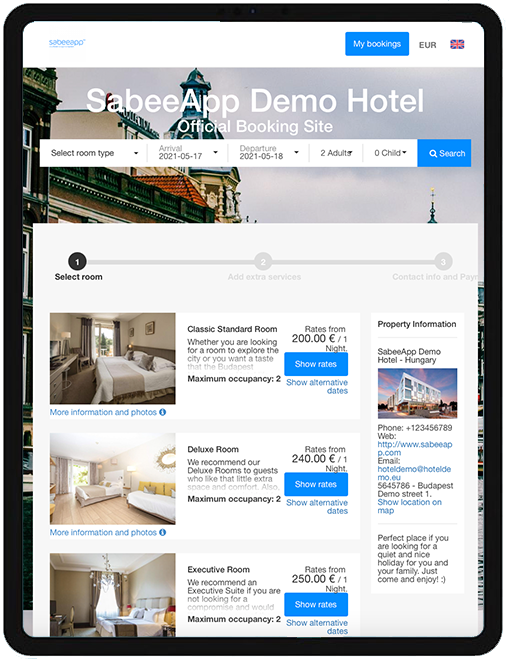This image showcases the official booking site of the Sabi App Demo Hotel. At the top, a clean, white banner spans across the screen, prominently featuring the Sabi App logo in blue on the left side. To the right, a blue "My Bookings" button is visible next to a "Europe" label. Directly beneath this banner, there is an intricate image capturing the ornate roof of an elegant building. Overlaid on this image in white text is "Sabi App Demo Hotel" with "Official Booking Site" just below it. 

Another white banner stretches horizontally across the page below, allowing users to select room types, arrival and departure dates, the number of adults, children, or to initiate a search. Below this functionality, the page displays a vertical list of various room options, complete with pricing details and interior images of each room, providing potential guests with a comprehensive overview of their lodging choices.